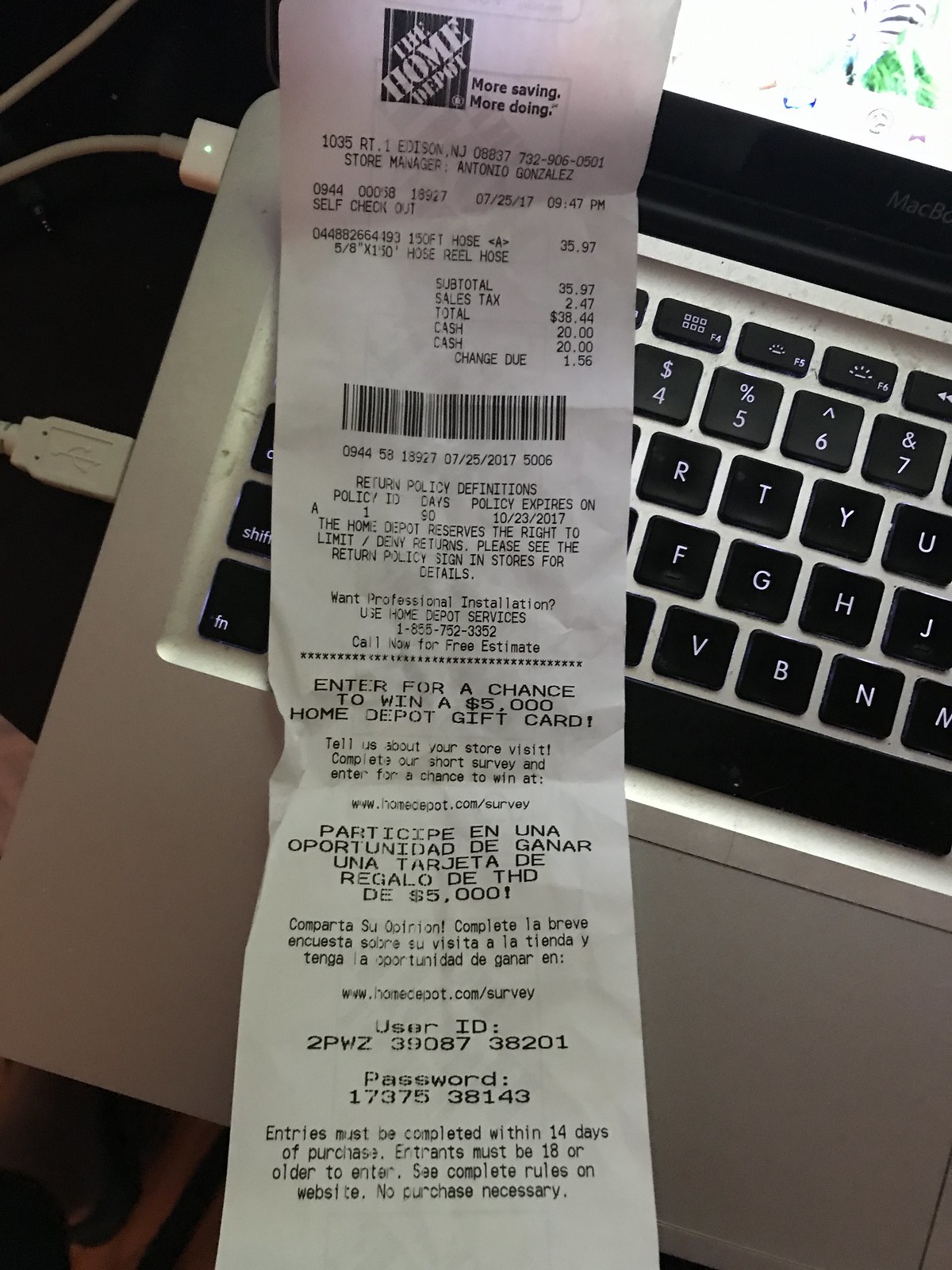The image captures an overhead view of a very long Home Depot receipt resting on the keyboard of a silver laptop. The receipt, with its distinct Home Depot logo visible at the top center, is slightly creased, causing it to angle up prominently. Printed with black ink on white paper, the receipt showcases a large rectangular barcode positioned centrally. Toward the bottom, there are phone numbers accompanied by a promotional message inviting customers to enter for a chance to win. The receipt lies at an angle, with its top portion located at the top left of the keyboard and its bottom portion toward the center. The laptop features black keys with a gray touchpad beneath the keyboard. Additionally, two white cords are plugged into the left side of the laptop, contrasting with the silver body of the device.